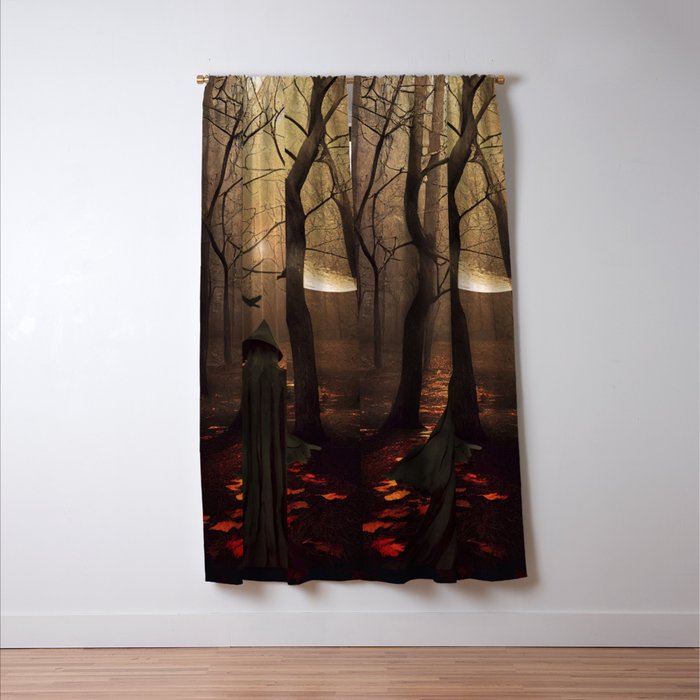This image showcases a set of artistic curtains hung on a six-pane window against a white wall, with a black curtain rod at the top. The curtains display an eerie woodland scene at sunset. Central to the image is a sinister figure resembling an old wicked witch, clad in a gray robe and a pointed hat, walking into a sparsely populated forest clearing. The leafless trees depicted on the curtains provide a stark backdrop, while red leaves scattered on the ground hint at autumn. Birds are seen flying over the witch's head, creating a dynamic element to the scene. The setting sun, whose yellow light is gently filtered through the trees, and a quarter moon appear prominently in the design, adding to the mysterious and slightly ominous ambiance. Aimed to strike a balance between the ethereal and the creepy, the detailed elements on the curtains combine with the structure of the window to create a captivating visual narrative.